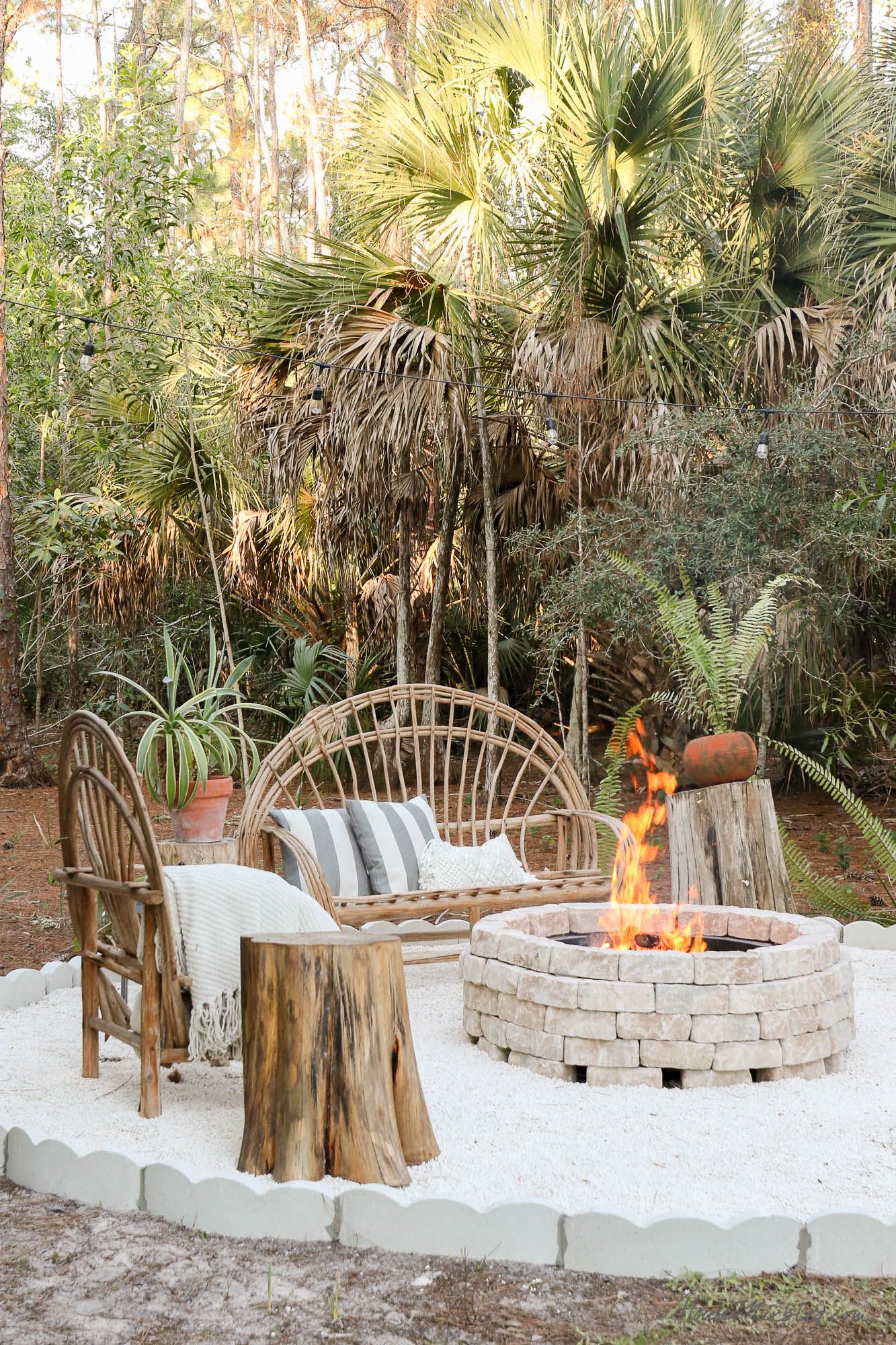In this outdoor daytime scene, the image showcases a cozy sitting area centered around a fire pit made of white bricks, which sits on a white concrete platform bordered by white stones. This stylish, photographic image subtly combines various earthy tones and inviting textures. The fire pit, with a visible flame, is slightly off-center to the right. Surrounding it is a harmonious arrangement of furniture: a brown curved-back rattan loveseat adorned with two gray and white pillows, and a thin white pillow stands directly behind the fire pit in the center. To the left of the fire pit is a wicker easy chair draped with a blanket, next to a grayish-brown tree stump that serves as a rustic side table. The sitting area is encircled by a small barrier containing a sandy patch, adding to its beachy, relaxed vibe. The background is decorated with verdant palm trees and other plants, enhancing the natural feel of the setting. The overall palette of the image includes shades of brown, gray, blue, red, yellow, green, and a hint of orange, all contributing to the serene and inviting atmosphere. The scene has no text, focusing entirely on the tranquil ambiance of this charming outdoor retreat.